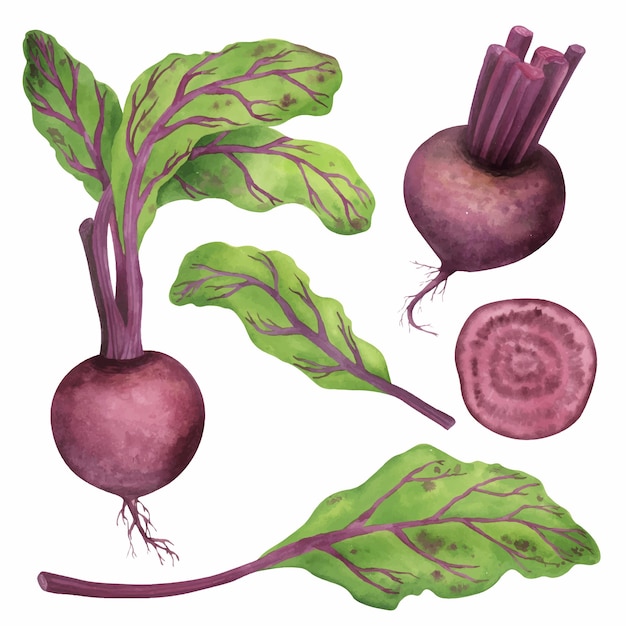The image is a watercolor painting with a white background, depicting various aspects of a beet or beetroot. On the left-hand side, there's a complete beetroot showing the full bulb at the bottom, with small root branches and a purple stalk that has green leaves with purple veins. The bottom of the picture features a single beet leaf with a stem. In the center of the image, there's another smaller beet leaf. The top right-hand corner shows a beetroot with its leaves cut off, leaving only the purple stems. Below this, in the middle right section, there's a cross-section of the beetroot, illustrating its dark burgundy-purple rings. The beetroot itself is a rich red or purple color, harmonized with the green and purple hues of the leaves and stems.